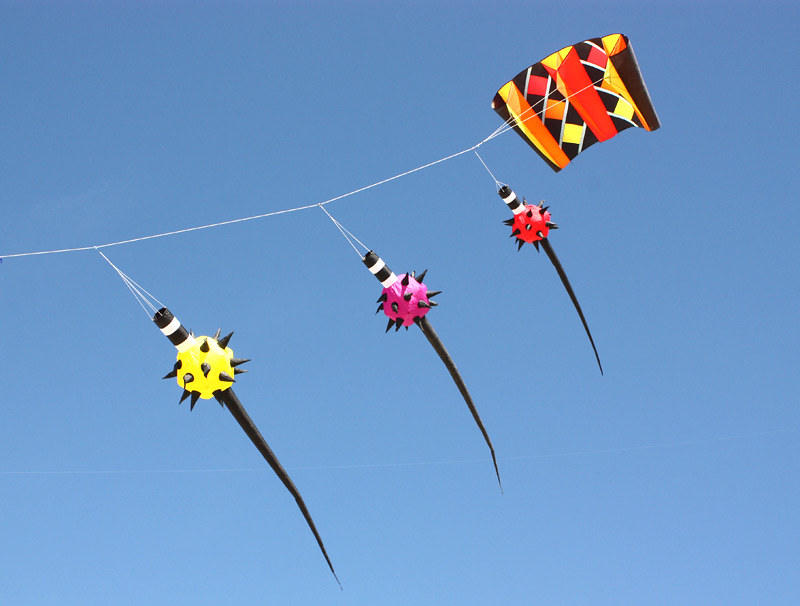This photograph captures a vibrant scene of a striking kite soaring in a cloudless, deep blue sky. Dominating the image is a large kite with a distinctive design: it showcases black edges framing an eye-catching red stripe down its center, flanked by vivid orange on the left and bright yellow on the right. The kite’s surface features a pattern of diagonal white lines, which intersect to create diamond shapes – red, orange, and yellow – adding a dynamic, geometric flair to the overall design.

Three smaller, cylindrical kite-like objects are tethered to the main kite's string, each suspended by its own offshoot line. These objects are vividly colored in red, purple, and yellow, each adorned with menacing black spikes and a tapering black tip. Their striped cylindrical sections alternately display black and white bands, culminating in pointed cone-like tails. The yellow object has three strings, the purple has two, and the red features four strings, contributing to the intricate and colorful aerial display.

Overall, the photograph brilliantly captures the lively and detailed assemblage of kites against a crisp, clear sky, with intricate designs, vibrant colors, and dynamic forms creating a visually captivating scene.